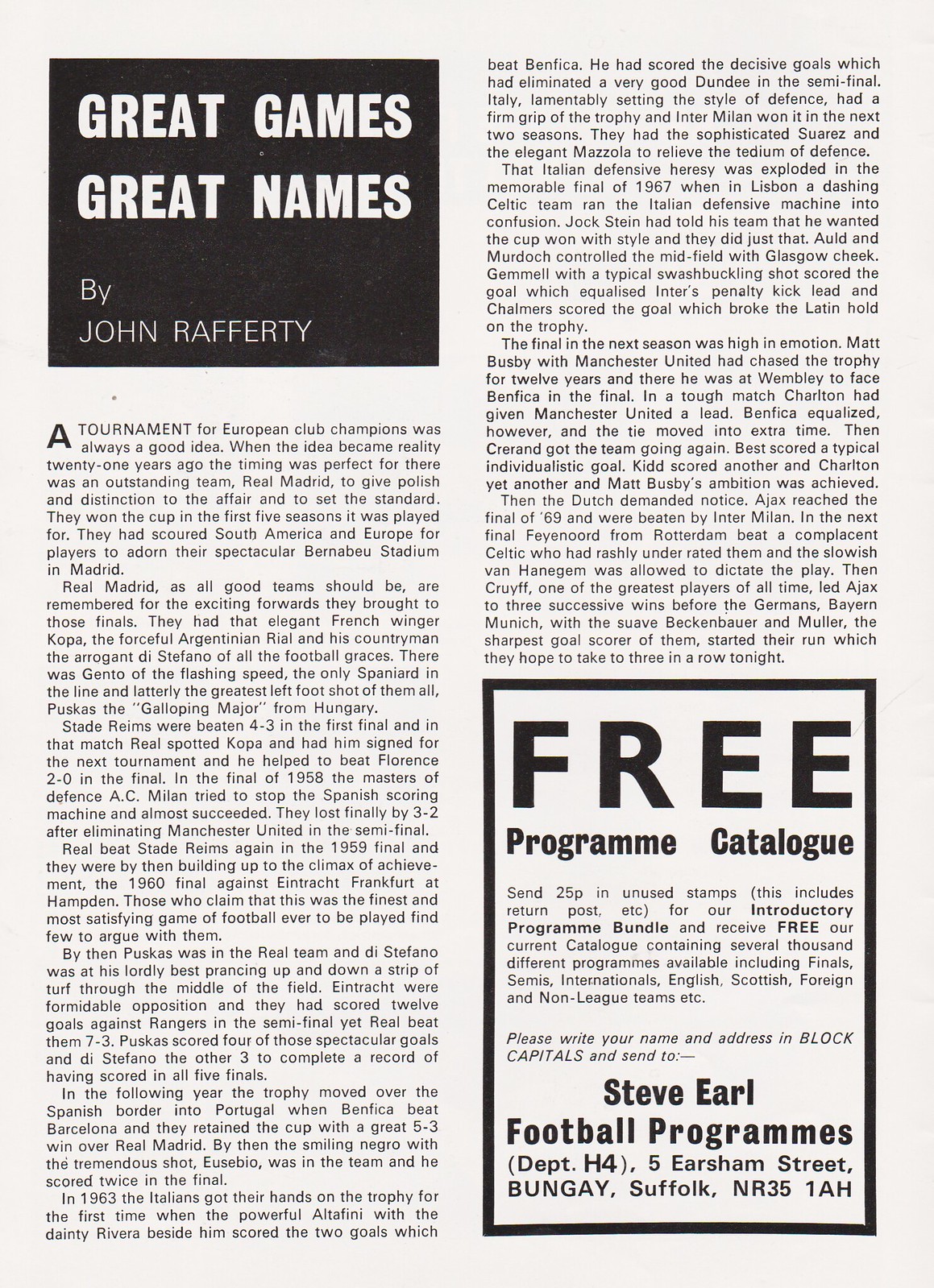This image depicts a vintage magazine or newspaper article from the mid to late 1960s to early 1970s, printed on an off-white sheet of paper. The article is titled "Great Games Great Names" by John Rafferty, prominently displayed in white block capital letters within a black box in the upper left corner. The content is organized into two columns of black text that narrate the enduring appeal and history of European club championships, detailing the tournaments and their celebrated trophies over the years.

Towards the end of the article, there is an advertisement bordered by a tall black rectangle in the lower right corner. The ad, emphasizing prominently the offer “Free Program Catalog” in black capital letters, invites readers to send 25 pence in unused stamps to receive a program bundle. This bundle includes a catalog featuring thousands of programs from finals, semis, internationals, and various leagues including English, Scottish, foreign, and non-league teams. The address provided for the response is to Steve Earle Football Programs Department, at H45 Ersham Street, Bungay, Suffolk, NR351AH. Overall, the article and the advertisement are laid out neatly from the top left to the bottom right of the page against a light beige background, creating a comprehensive and engaging read for sports enthusiasts.